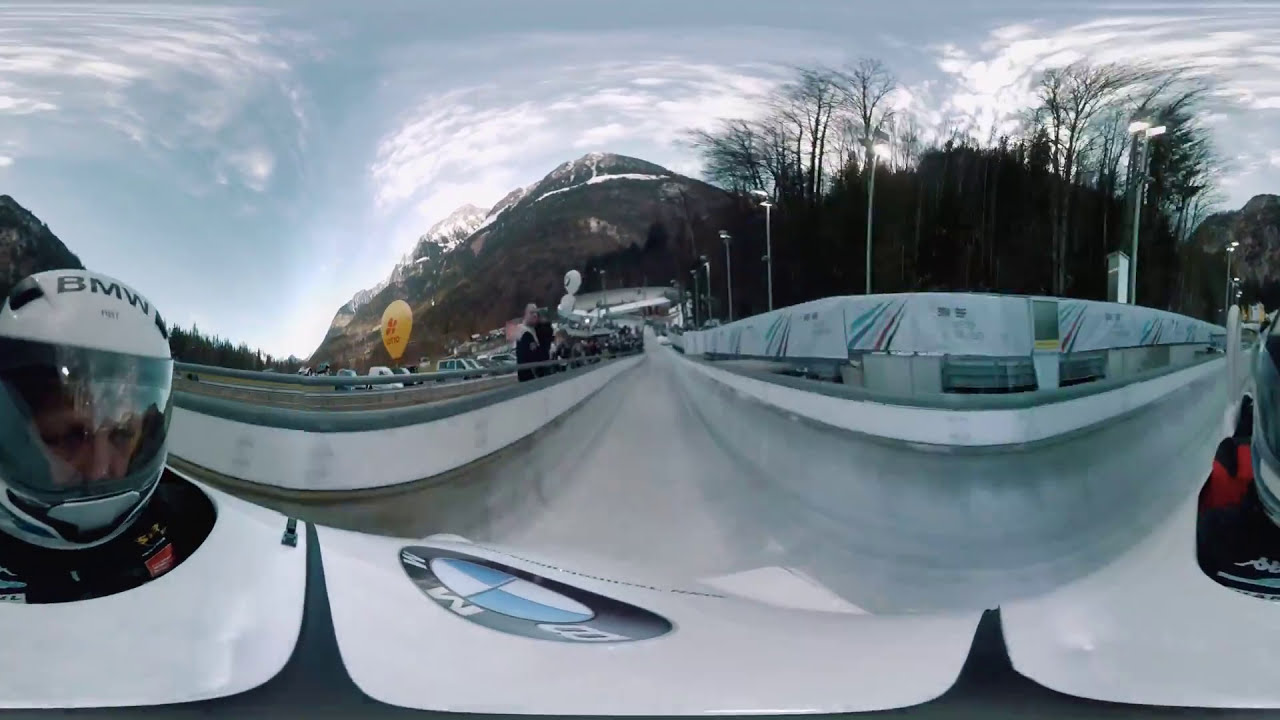The photograph captures a dynamic moment of a bobsledding event, possibly an Olympic competition, set against a breathtaking mountainous backdrop. The image is slightly distorted due to the camera's wrap-around perspective. In the foreground, a bobsledder, positioned at the front of a sleek BMW-branded bobsled, is clearly visible. The athlete is donned in a white helmet prominently featuring the BMW logo, a circle segmented into blue and white quarters. The bobsled itself is primarily white with black accents and a hint of red at the bottom, also bearing the iconic BMW emblem. The icy bobsled track curves through the scene, emphasizing the speed and intensity of the sport. In the background, towering, snow-capped mountains and a partly cloudy sky frame the setting. Signage in an Asian language suggests the location might be in a Chinese or Japanese region. Spectators are seen along the left side of the track, intently watching the thrilling descent.